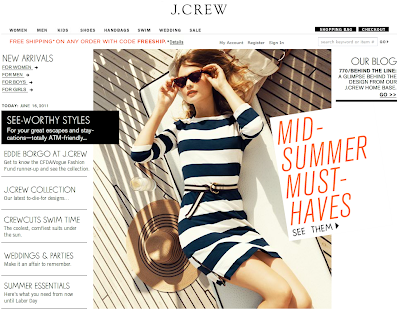**Fashion Website Overview: J.Crew Home Page**

At the top of the fashion website, centered prominently, the logo "J.Crew" is displayed. On the left side under the logo, there are several clickable buttons in black. These buttons include categories labeled "Women," "Men," an obscured label, "Shoes," "Handbags," "Swim," "Wedding," and "Sale."

In the center, the main image features a female model lounging against a neatly made bed with white linens bordered in black. Her tan hat, adorned with black spirals converging to the center, lies on the floor nearby. The surface she's laying on has sections of both white and brown. The model is wearing black shades with dark brown temples and tops. Her dirty blonde hair, cascading gently around her face, reaches shoulder length. She sports a stylish, light-skinned complexion with a white dress adorned with dark blue stripes. The image suggests a sunny day.

On the right side of the image, additional content reads "Our Blog" and a section marked with "TTG behind the line," suggesting behind-the-scenes content from J.Crew's design team. Beneath this, a partially visible rectangle in orange reads "Midsummer Must-Haves," with further prompts to "See Them" in black text below.

Directly underneath the top navigation bar, highlighted in orange, there's a promotional offer: "Free Shipping on any order with code FREESHIP," with "Details" underlined in black.

Below the main promotion, further navigation options appear. These include "My Dashboard," "Register," and "Sign In." Further categorization is visible, with sections for "New Arrivals," "FDR Women," "PGR Men," "FDR Boys," and "PDR Girls." Additionally, there is a rectangle with a black background featuring white text: "Sea-Worthy Styles," followed by bold white text stating "For Your Great Escape." Due to blurring, the following text is partially unreadable.

The left navigation also includes mentions of "Eddie Borgo at J.Crew," the "J.Crew Collection," and themes like "Crew Cuts," "Swim Time," "Weddings and Parties," and "Summer Essentials."

This detailed layout offers a comprehensive view of J.Crew's product lineup and special promotions, enhancing the online shopping experience for visitors.